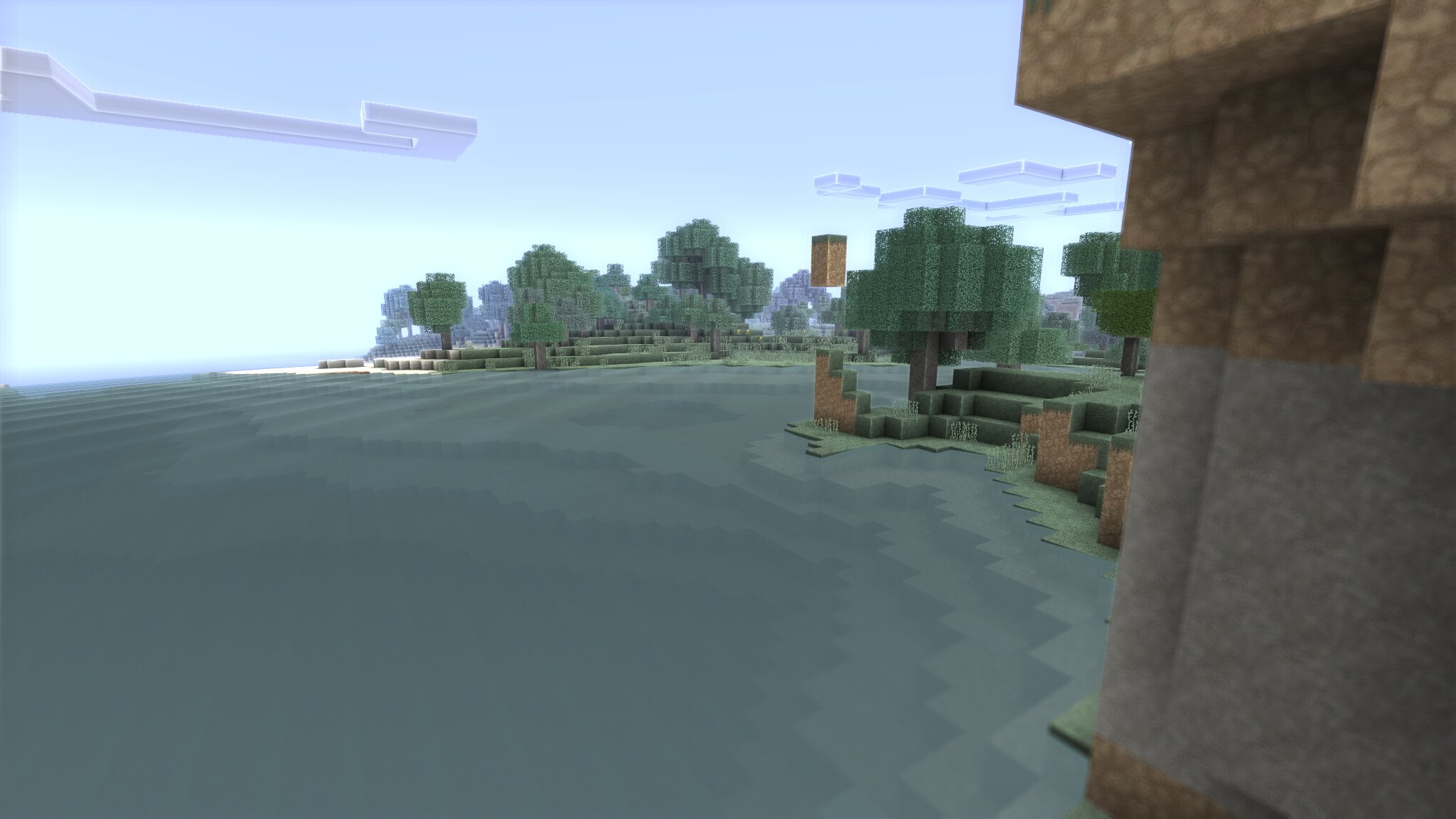In this image, we see a detailed and vibrant Minecraft world. The landscape is unmistakably from the video game Minecraft, characterized by its pixelated, blocky appearance. In the foreground on the right, there are close-up reddish-brown and grayish-brown bricks that enhance the scene's textured depth. The ground is covered with green grass and patches of red-brown dirt, leading to an angled slope that ascends from the shoreline. 

The scene features the expansive sea, depicted in a deep, yet somewhat faded blue hue, with a rocky underwater terrain that hints at the depth of the ocean. To the left of the image, the sea contrasts with the land and adds a sense of vast space to the composition.

Dotting the shoreline and extending into the distance are numerous trees, constructed from dark green blocks. These trees have no visible branches, emphasizing the game's unique aesthetic. Some trees in the background appear in shades of medium gray, adding to the diversity of the landscape. 

Floating above the terrain are various blocks and platform-like formations, contributing to the scene's whimsical and imaginative nature. The sky is mostly clear, populated by flat, rectangular clouds with various shapes within, executed in a blocky design that is signature to Minecraft.

Overall, the image captures a beautiful, clear day in the Minecraft world, blending the natural elements of a beach, ocean, and forest with the game’s iconic blocky, pixelated style.